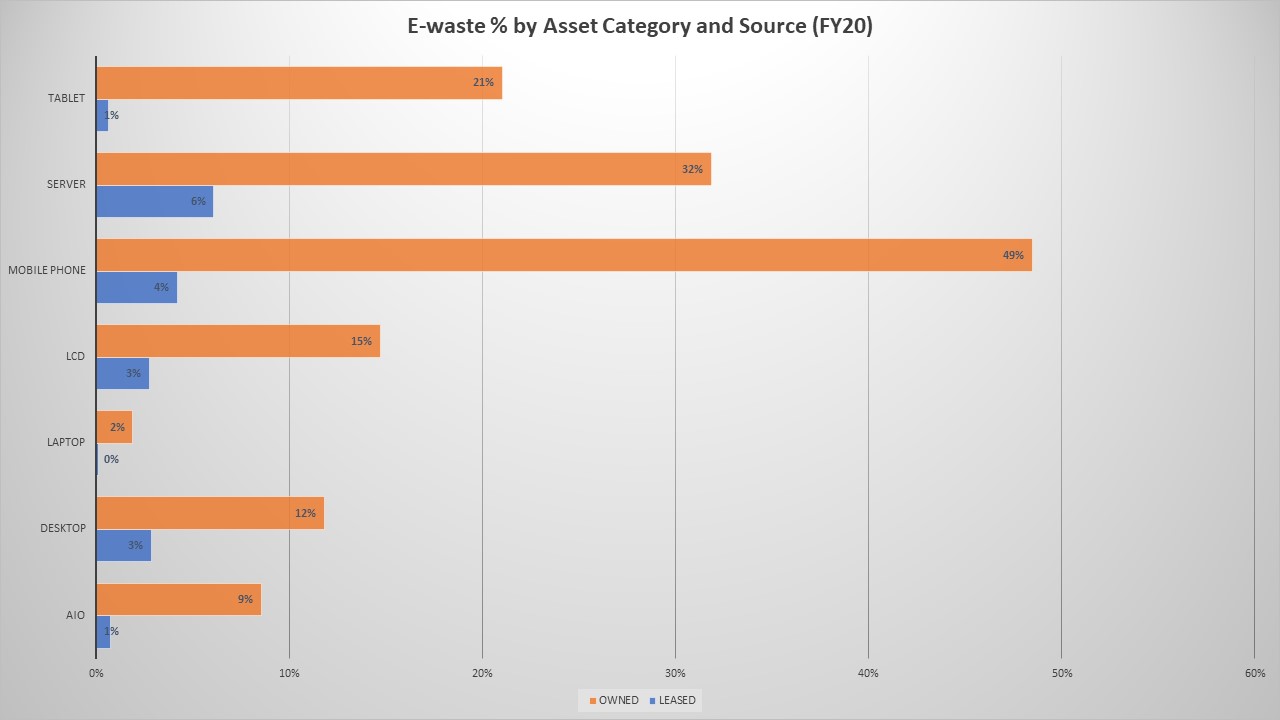The image is a rectangular, horizontal bar graph titled "E-Waste Percent by Asset Category and Source (FY 20)." The background is white, and the graph displays data separated into two categories: "owned" in orange and "leased" in blue. These categories are compared across various asset types, listed on the vertical axis as tablets, servers, mobile phones, LCDs, laptops, desktops, and AIOs. The horizontal axis, which ranges from 0 to 60 percent, represents the percentage of e-waste. Among the categories, mobile phones show the highest disparity, with 49% owned and 4% leased. In general, the graph indicates that a higher percentage of these electronic devices are owned compared to leased.